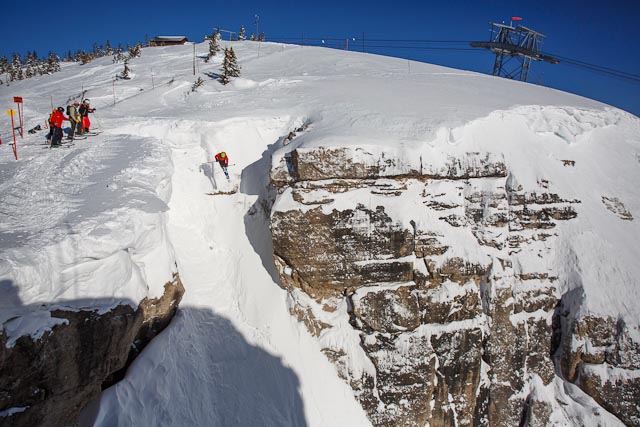In this captivating outdoor winter photograph, a dramatic ski slope extends steeply downward, enveloped in several feet of packed snow. A skier, donning a yellow helmet, red jacket, and blue pants, is courageously navigating the narrow, snowy passageway between two rocky cliff faces. His ski poles are poised as he makes his descent. To the left of the skier, three individuals stand closely together, eagerly awaiting their turn, their anticipation palpable. The scene is further adorned by a few colorful markers—a red and a yellow pole—embedded in the snow. In the distance, a majestic backdrop of snow-covered trees and a blue sky contrasts beautifully with the rugged terrain, while at the top, a ski lift is faintly visible against the intense azure, alongside a small cabin nestled among the trees. This image encapsulates the thrill and beauty of high-altitude skiing amidst a breathtaking winter landscape.